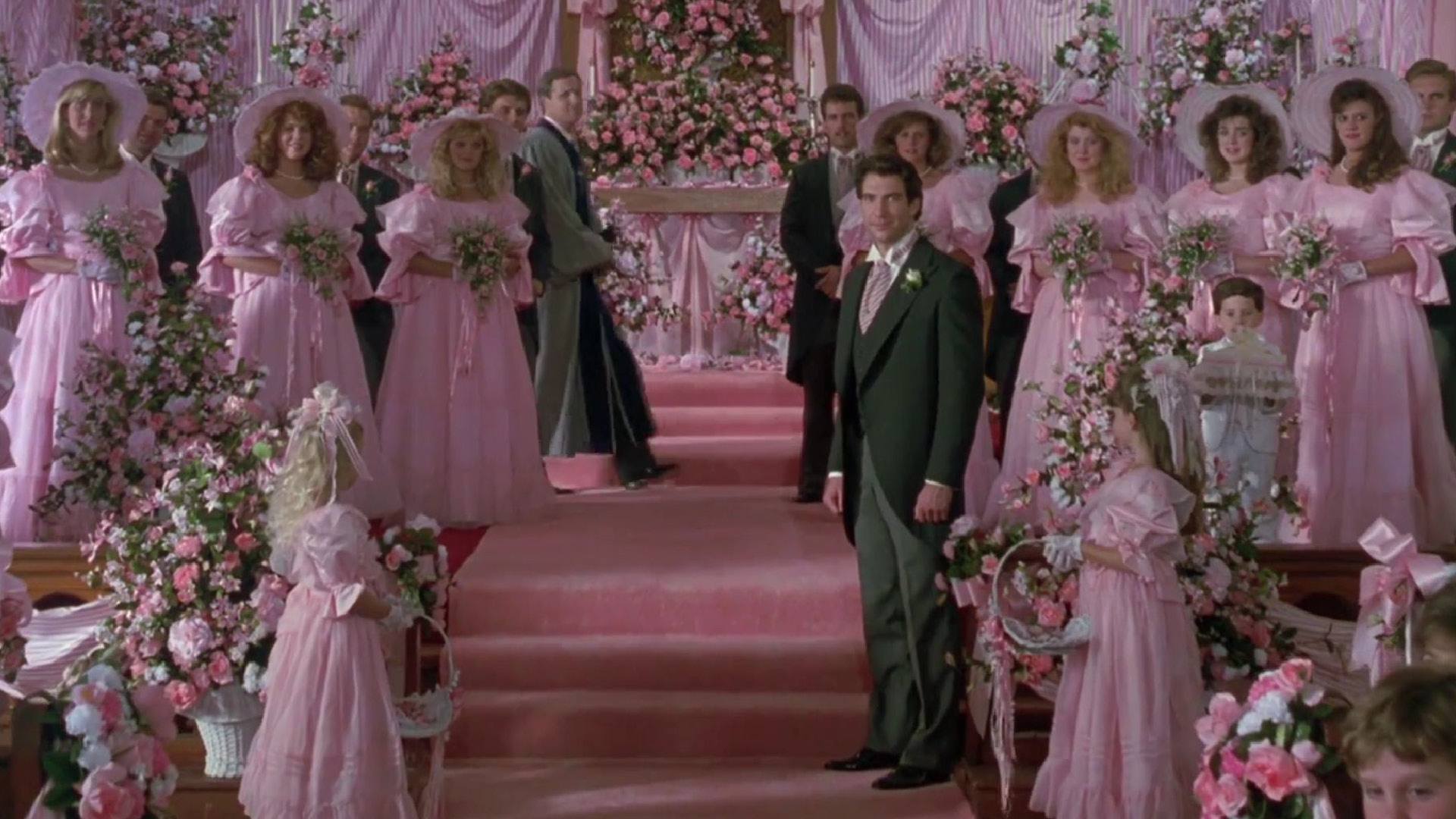In this wedding scene, the predominant color is pink, adorning virtually every element. Central to the image is an altar lavishly decorated with pink flowers and greenery, standing before a backdrop of pink curtains and floral arrangements. Flanking the altar are groups of women, with three on the left and four on the right, all wearing coordinated pink dresses and pink hats, each holding pink floral bouquets. A striking pink carpet stretches down the walkway, leading up to the steps of the altar, also covered in pink rugs.

On either side of this carpet, two young girls in matching pink outfits stand, holding small baskets, adding to the coordinated pink theme. A man in a crisp suit, possibly the groom, stands on the first step of the staircase, looking towards the center. In the background and towards the altar, several men in tuxedos are seen, including one in a lighter gray tuxedo, who might be the officiant or another key figure in the ceremony. A young boy dressed in white is also visible near the center, providing a contrast to the pink attire of the bridesmaids and the general decor. The entire scene is a harmonious blend of pink, with floral elements and meticulously arranged participants, creating a visually striking and cohesive wedding tableau.